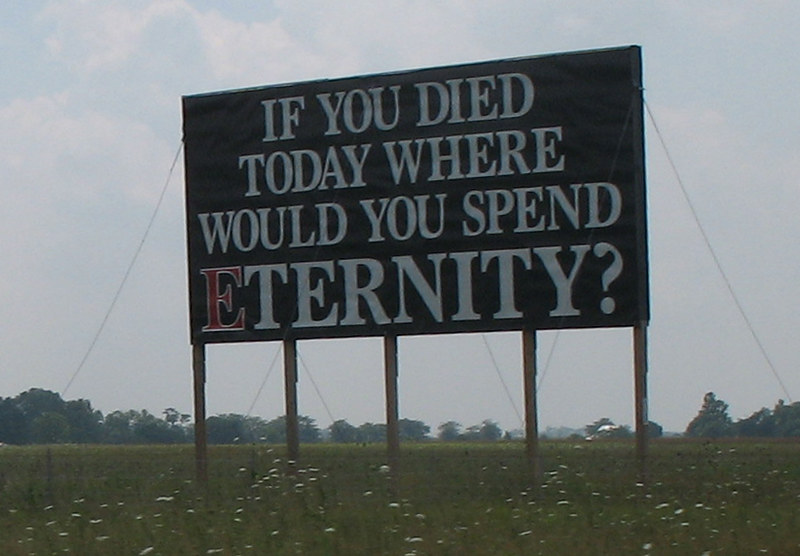The photograph depicts a large, rustic wooden billboard situated in a grassy field filled with tall, white, daisy-like flowers and Queen Anne's lace. The sign, which is supported by several posts and wires for stability, prominently displays the message: "IF YOU DIED TODAY, WHERE WOULD YOU SPEND ETERNITY?" The lettering is mostly in white capital letters, except the first letter 'E' in "ETERNITY," which is strikingly highlighted in red. The background of the sign is black, creating a stark contrast that emphasizes the message. In the distance, you can see a scattering of large trees and possibly a farm structure like a house or barn. The sky above is overcast with clouds, though a peek of blue is visible in the upper left-hand corner, suggesting it is a cloudy yet bright day. The scene appears to be from an older photograph, adding a nostalgic quality to the rural landscape. This imagery suggests a reflective, possibly religious prompt about life and the afterlife, common in church or salvation-themed messages.